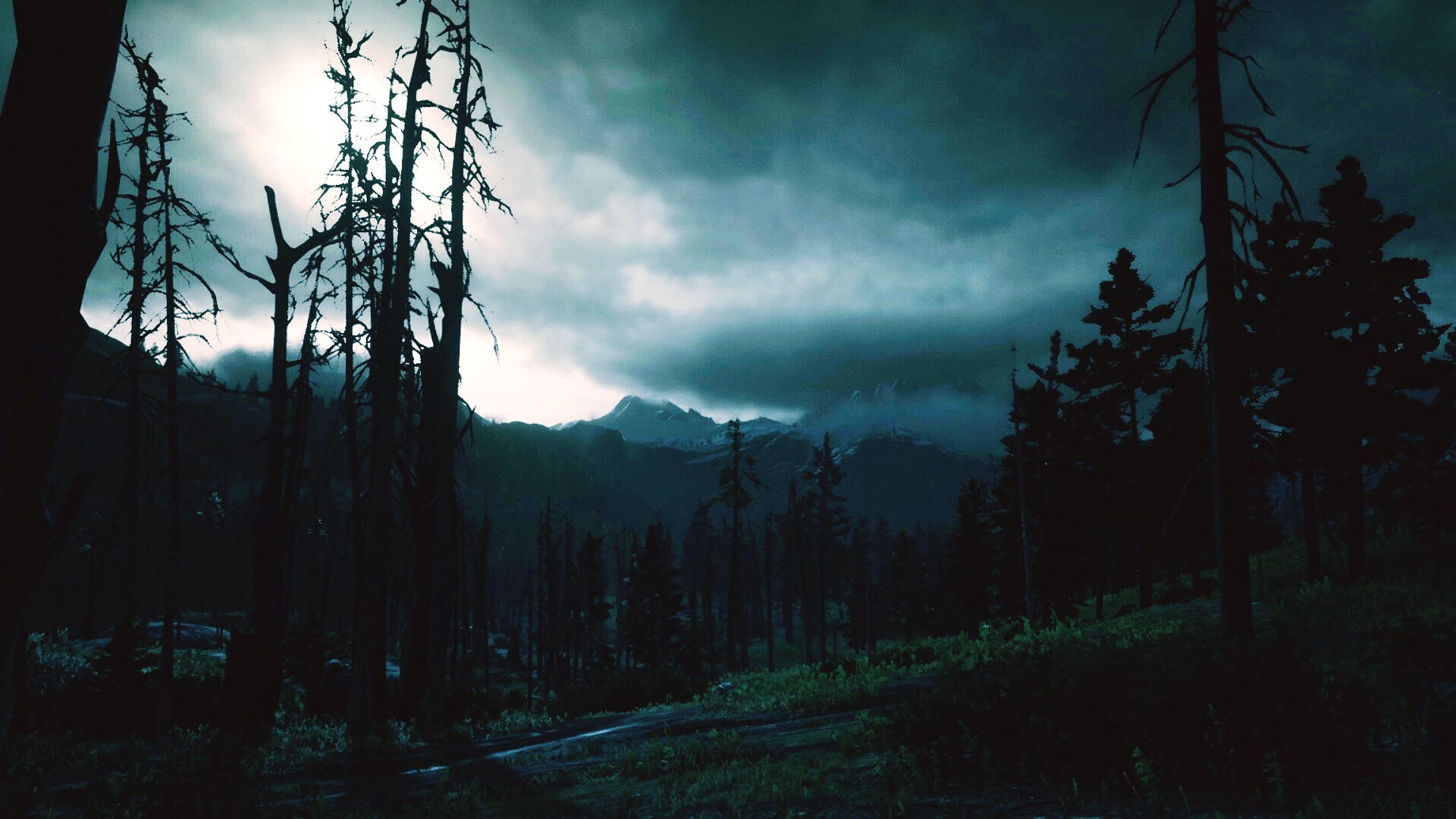This captivating painting showcases a somber, twilight scene with a range of delicate details. In the foreground, a gently sloping hill blanketed in grass stretches out, interrupted by smooth, slippery rocks that catch the faint gleam of moonlight. Tall, leafless trees with bare branches dominate this area, their stark silhouettes adding to the scene's melancholic atmosphere. 

Transitioning to the mid-ground, a dense cluster of evergreen pine trees stands as a dark, reassuring presence. Beyond them, a craggy mountain range towers in the distance, its snow-capped peaks shimmering subtly under the muted lunar glow.

Above, the sky is cast in heavy, dark gray clouds, creating a somber, overcast ambiance. Despite the oppressive cloud cover, the moon endeavors to pierce through, casting ghostly patches of light that dance across the landscape, reflecting off both the dew-kissed grass and the slippery rocks. The overall depiction exudes an eerie, yet serene beauty, capturing a tranquil moment teetering on the edge of night.